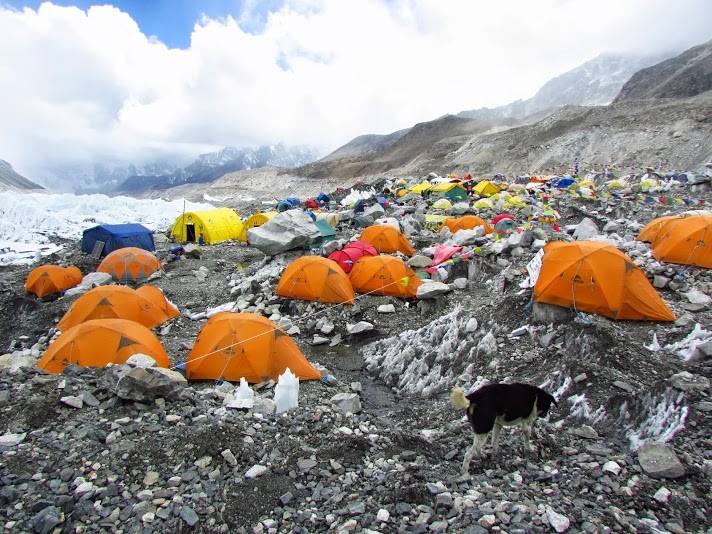The image depicts a sprawling mountain campsite set in a cold, rocky terrain, likely high in the mountains. The area is filled with at least 50 colorful tents, with many of the ones closest to the camera in shades of orange while those further back display a variety of colors, including yellow, blue, red, white, gray, green, and pink. A glacier appears to be visible on the left side, contributing to the icy and stony landscape that rises up to meet cloudy mountaintops in the distance. The sky is mostly overcast with a patch of blue peeking through in the top left corner. Scattered about the campsite, thin string lines can be seen running between the tents, and near the camera, there is an animal, possibly a goat, interacting with the icy rocks. The scene is devoid of people, suggesting it might be a base camp for a mountain climbing expedition.